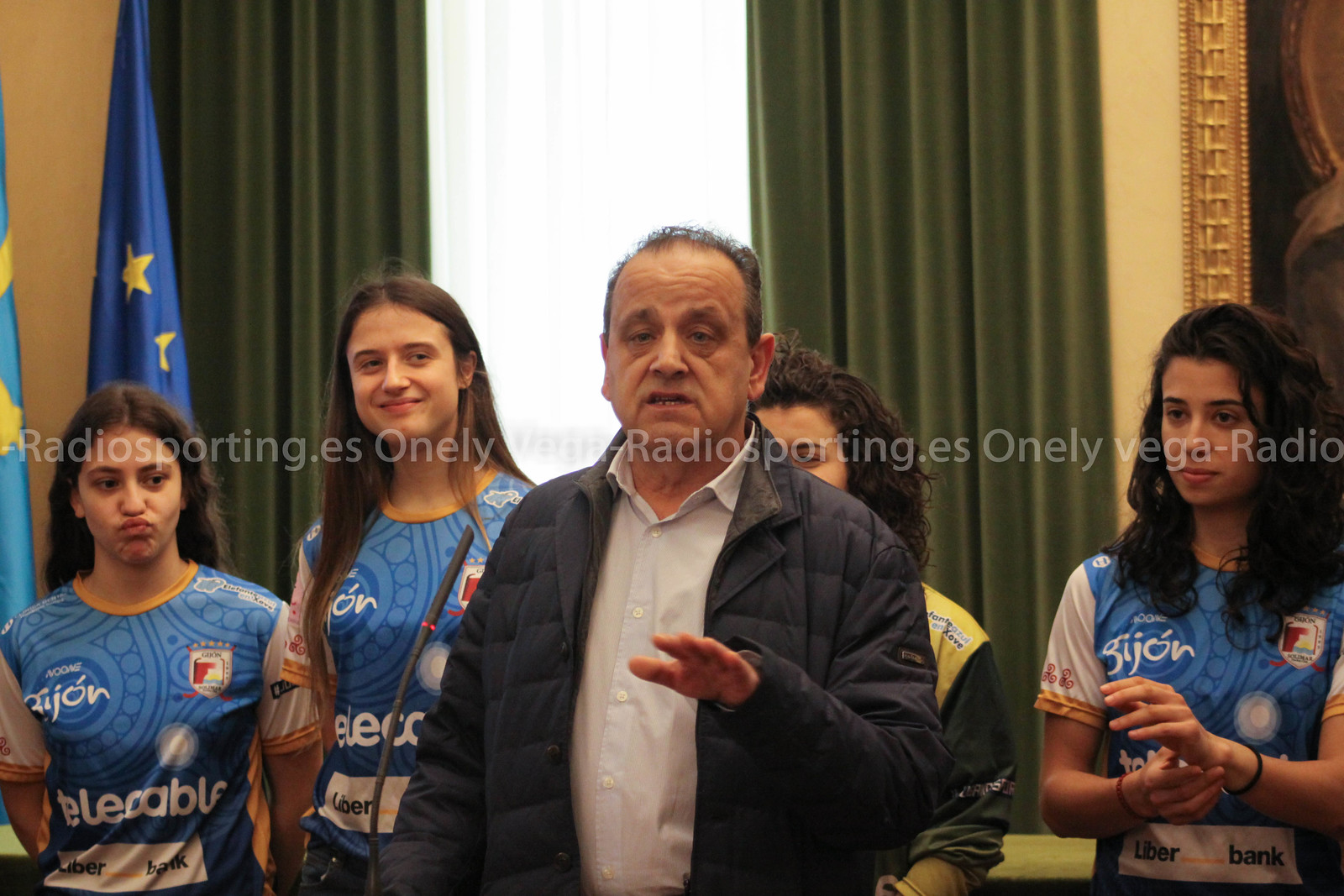This photograph captures a moment where an older man with receding dark hair, dressed in a dark blue or black jacket and a white button-down shirt, is centered in the image as he speaks with his right hand held in front of him. The man, who appears to be in his 50s or 60s, is standing in what looks like a fancy office. Behind him stand four young women, all with long dark hair, wearing matching blue and white shirts or jerseys adorned with various logos and white writing, possibly for a sports team. The women, seemingly teens, have their eyes on the man, creating a focused and attentive backdrop. A window flanked by large green curtains occupies the center of the background, its yellowish-golden walls adding a warm tone to the scene. On the left side, two flags in shades of blue and yellow stand upright but are not unfurled, hinting at their significance. The detailed setting and organized appearance of the group suggest this could be a team event, possibly with the coach addressing his players.